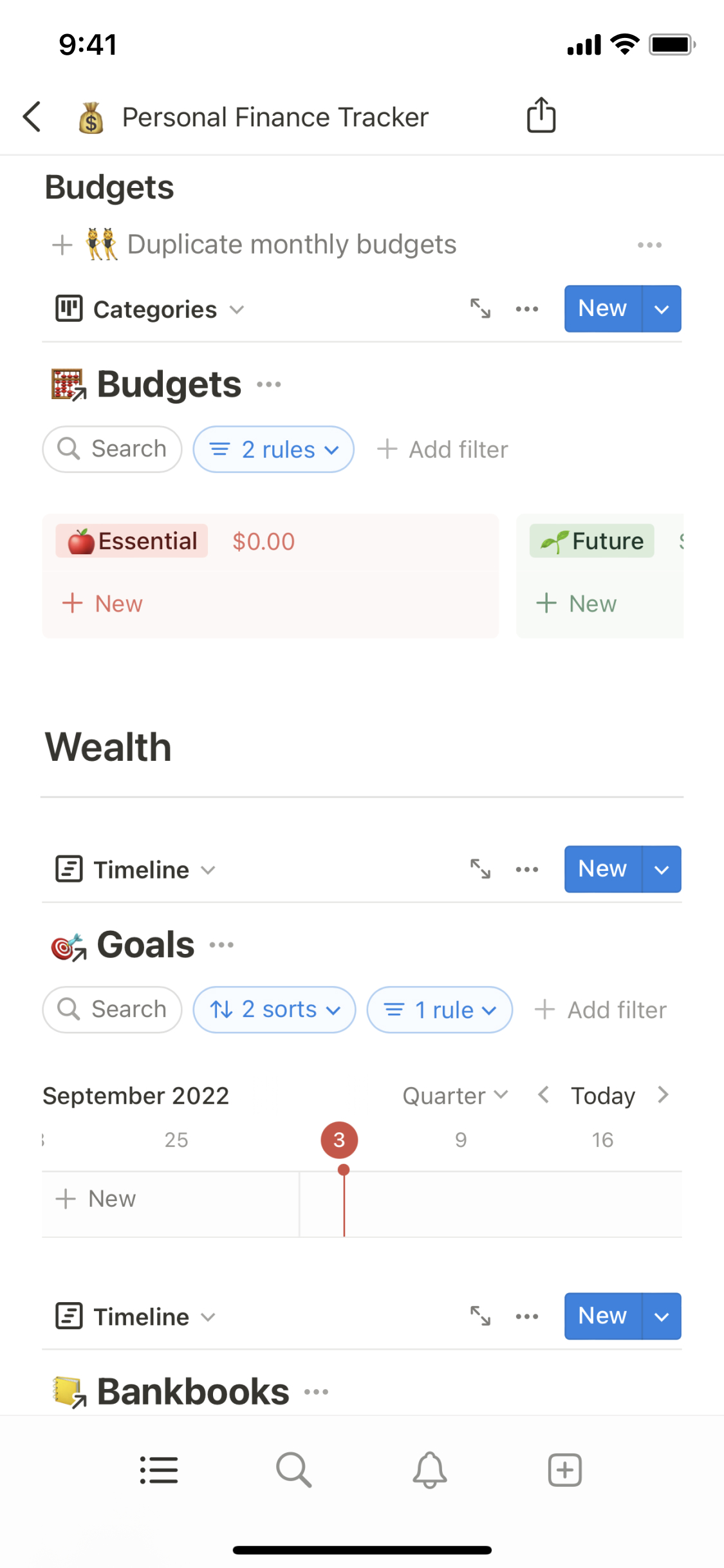The image is a screen capture from a tablet displaying an app for Personal Finance Tracker. The time displayed at the upper left corner of the screen is 9:41. The device shows full telephone signal, full Wi-Fi connectivity, and a fully charged battery.

The app interface is titled "Personal Finance Tracker," situated at the top center of the screen. Below this, a navigation section labeled "Budgets" is visible. There is also a plus sign icon accompanied by the text "Duplicate Monthly Budgets," and a drop-down arrow indicating additional categories under the budget section.

Next, there appears another "Budgets" section marked with a red calendar icon to its left. This section includes a "Search" icon, two "Rules," and an "Add Filter" option. Below this is a category titled "Essential," represented by an apple icon, showing a balance of $0.00. There is a plus sign next to this section to add new data.

To the right of the "Essential" section is another category named "Future," symbolized by a plant icon. This section also features a plus sign to add new data. Thus, the primary navigation under "Budgets" comprises the "Essential" and "Future" categories.

Following the budget metrics, is a "Wealth" section. Inside this section, there are options labeled "Timeline," "Goals," and relevant menu options. The "Timeline" feature has a drop-down menu, while the "Goals" feature includes a "Search" icon, two "Sort" arrows, an option for one rule with a drop-down menu, and a plus sign to add a filter.

Below these sections, there is a calendar for September 2022. The calendar starts from the 25th, with particular dates like the 3rd highlighted in red. It appears to show a sequence of weeks, with dates such as the 9th and the 16th marking specific weeks. There is also a selection for the current quarter and an option labeled "Today."

At the bottom of the app interface, another "Timeline" option is available with a drop-down menu adjacent to it. Further down, there is a section labeled "Bank Books," which includes various icons for a menu of selections, search functionality, notifications, and a plus sign for adding new data.